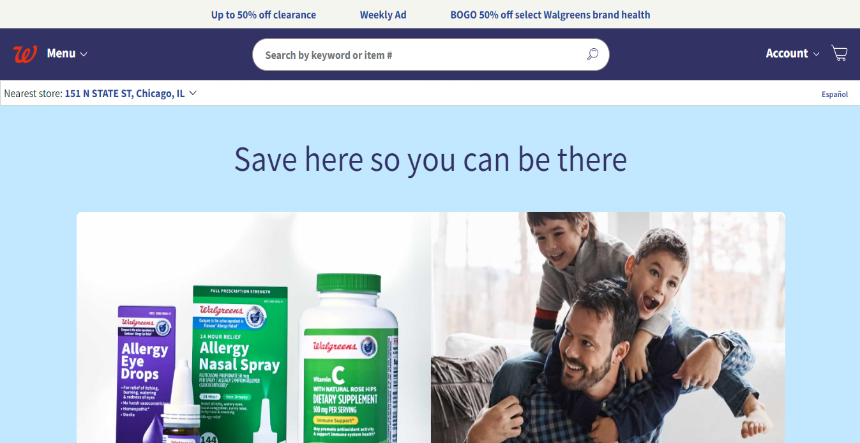The image features a computer screen displaying the Walgreens website. At the top, a light gray bar announces various promotions including "Up to 50% Off Clearance," "Weekly Ad," and "Buy One Get One 50% Off Selected Walgreens Brand Health." Below that, a dark blue band prominently features a red Walgreens "W" logo. To the side, there's a dropdown menu. Centrally located is a search bar that reads "Search by keyword or item number." Beside it, there are icons for account access with a dropdown menu and a shopping cart.

Beneath these elements is a white section labeled "Nearest Store," which includes a dropdown menu for selecting locations. Small print on the right side of this white bar indicates the availability of a Spanish-language option with the text "Español."

The main section of the screen headline, "Save Here So You Can Be There," is in bold lettering, followed by images of allergy medicine and vitamin C. Additionally, a boxed photograph depicts a joyful family scene: a father playfully wrestling with two boys who are sitting on his shoulders. They are all seated on a brown chair in a home setting, smiling and sharing a happy moment.